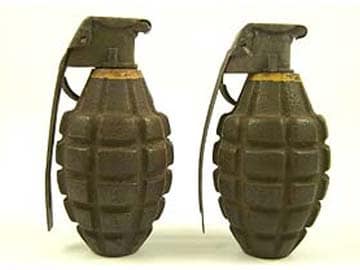The image depicts two identical hand grenades placed on a plain white surface with subtle shadowing beneath them. Both grenades are dark green, resembling the classic army green or olive color, with distinctive oval shapes similar to pine cones, marked by indentations. The top of each grenade features a flat surface that appears like a cap, adorned by a prominent gold or yellow band near the top. Extending to the left of each grenade is a long pin, likely used for detonation. The overall image is set against a plain white background and is somewhat blurry and of low resolution.